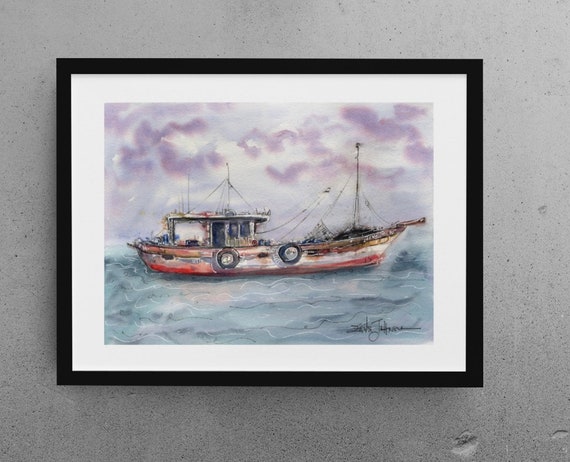The image displays a framed painting mounted on a light gray wall. The frame itself is black with a white border surrounding the artwork. The painting is a detailed depiction of a small ship navigating choppy blue-gray ocean waters under a purple sky. The ship, which could be a trawler, features a red bottom and a mostly white structure. It includes a single cabin, possibly the captain's quarters, with two windows and a door. The vessel also has an antenna and nets, and some lines attached to a pole at the front. The artist's autograph, written in black script, is visible at the bottom of the painting, though it is difficult to make out the signature.